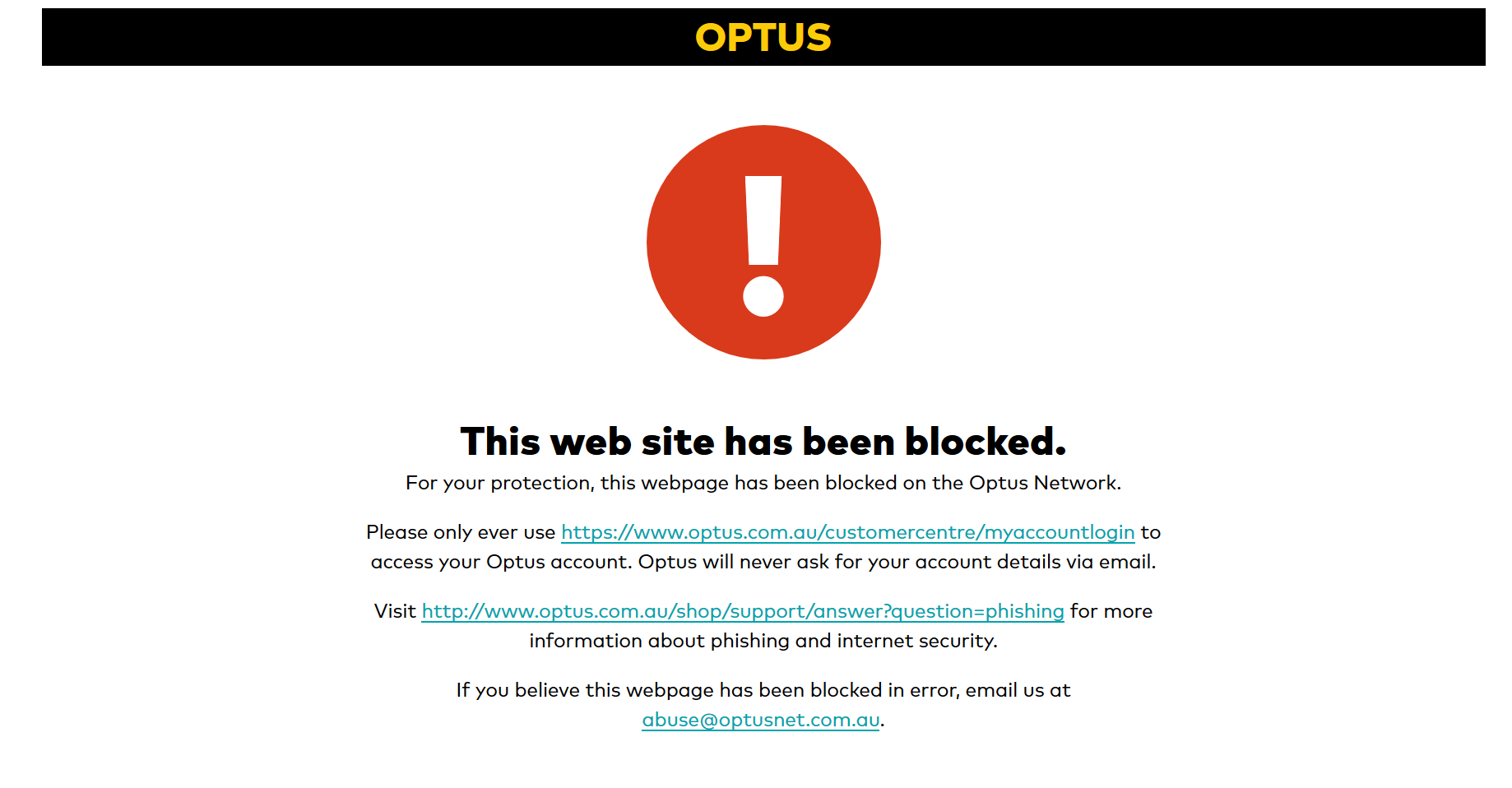The image features a stark white background with a prominent black rectangle displaying the text "Optus" in bold yellow letters. To the right of this, there is a striking red circle containing a white exclamation mark, drawing immediate attention.

Below these elements, a cautionary message is displayed in clear, readable text. The message states: "This website has been blocked for your protection. This webpage has been blocked on the Optus network. Please only ever use our official website (in blue) to access your Optus account. Optus will never ask for your account details via email."

The message continues with a recommendation: "For more information about phishing and internet security, visit our informational page (in blue)."

Finally, the image advises viewers on how to proceed if they believe the webpage was blocked in error: "If you believe this webpage has been blocked in error, please do not email us at abusc@optusnetwork.com.au." As a cautionary note, the email address "abusc@optusnetwork.com.au" is also highlighted in blue, indicating it's a clickable link.